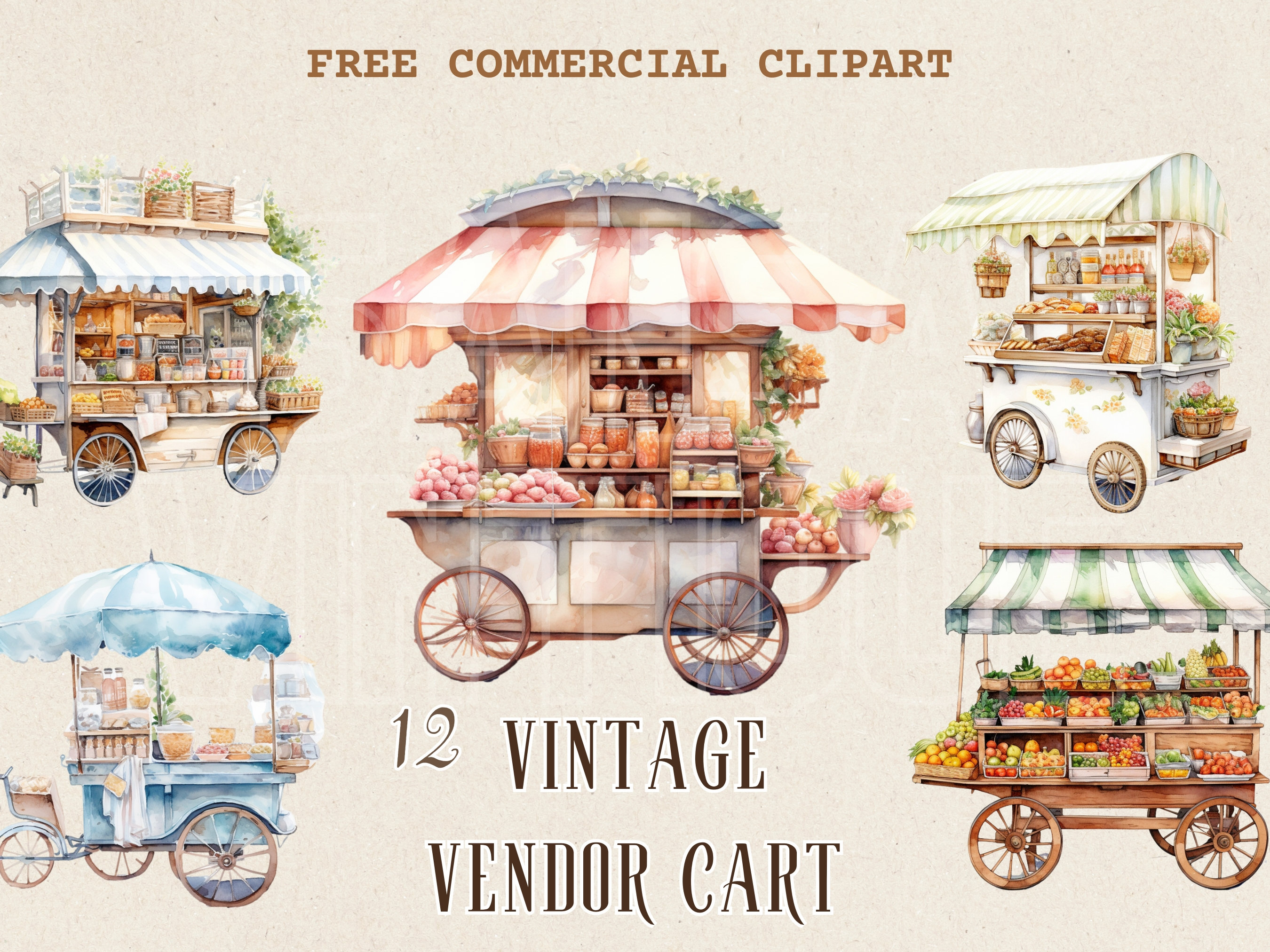A detailed collection of vintage vendor cart clip art, available for free commercial use, is featured at the top of the image. The bottom of the image labels this series as "12 Vintage Vendor Cart," although only five carts are displayed. Each cart is designed in an old-fashioned style with four wheels adorned with thin rims and multiple spokes, reminiscent of bicycle wheels. They are all open-air designs, equipped with awnings for shade and rain protection.

In the upper left corner, the first cart appears to sell an assortment of random food items. The cart in the middle showcases various jars and either fruit or potatoes beneath a red and white striped awning. Next to it, a cart with a yellow and white striped awning offers baked goods, some bottles, and several baskets filled with mixed vegetables. On the bottom row, the first cart seems to be selling iced tea stored in jars. The final cart features an array of fruits and vegetables, shaded by a green awning. The image offers an inviting glimpse into the nostalgic world of vintage street vending.